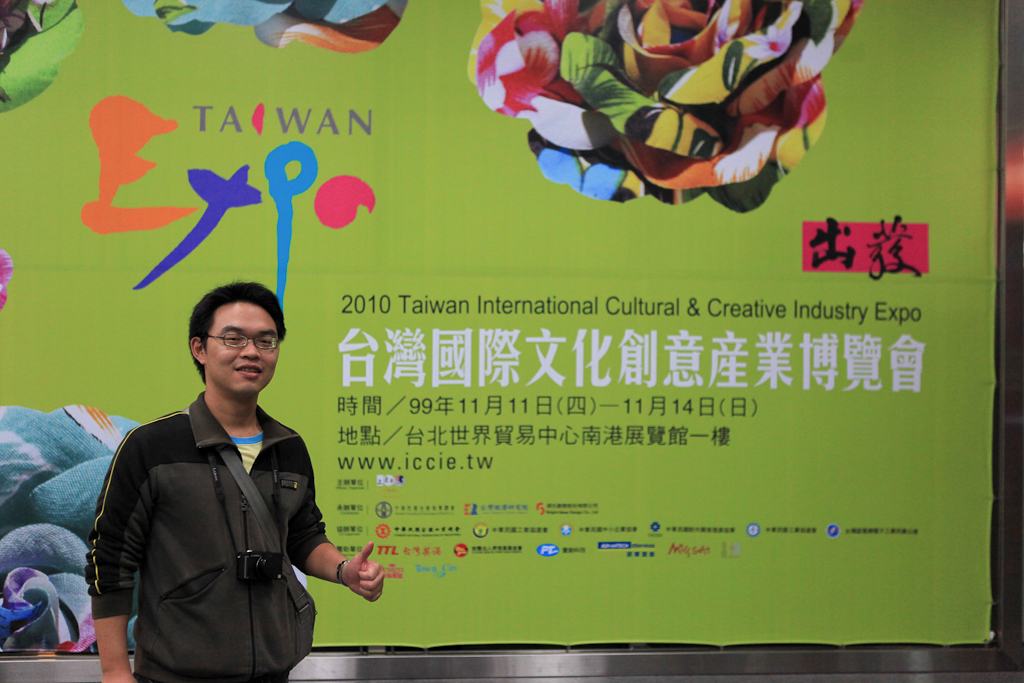In this image, a young Asian man, possibly in his late teens to early 30s, stands confidently in front of a large billboard, which serves as the entire backdrop. The man, located to the left side of the image and facing slightly to the right, has short black hair and wears glasses. He sports a gray jacket with black sleeves over a multicolored shirt, along with a camera hanging around his neck. With a cheerful demeanor, he gives a thumbs up with his left hand while his right arm rests at his side. The billboard behind him predominately features a light green background embellished with an array of multicolored designs, possibly floral or artistic elements. Prominently displayed at the top of the billboard are the words "Taiwan Expo," followed by "2010 Taiwan International Cultural and Creative Industry Expo" in English, with additional information in large white Asian characters and further inscriptions beneath. The man's cheerful expression and enthusiastic pose encapsulate the lively atmosphere of the event.